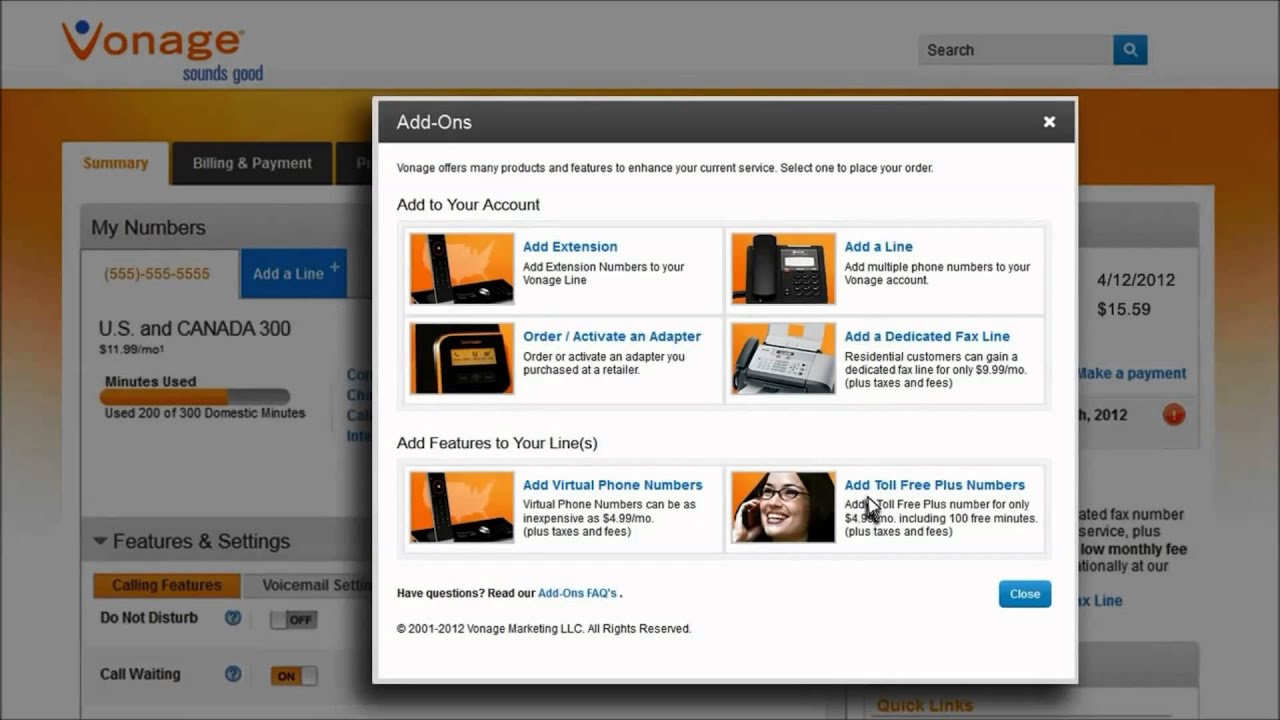The image captures a detailed screenshot reflecting a user interaction on the Vonage website, displayed on what seems to be a laptop or desktop screen.

### Background:
- **Header**: At the upper left-hand corner, there is the Vonage logo, featuring an orange capital "V" with a small blue dot above the letter. Beneath this, in small blue font, it reads "sounds good."
- **Search Bar**: Positioned on the right side of the header is a white search bar with the text "search" in black and accompanied by a blue box containing a white magnifying glass.
- **Website Navigation**: The faded gray background showcases various navigation tabs, such as "Summary," "Billing," and "Payment." The "Add-Ons" tab is notably selected, bringing its contents into sharper focus.

### Foreground:
- **Add-Ons Section**: 
  - **Header**: A black bar with the labeled "Add-Ons" in white text (formatted as "Add-Ons") heads the section. To its right is a small white "X" for closing the tab.
  - **Introduction**: Below this bar on a white background, a brief introduction reads, "Vonage offers many products and features to enhance your current service. Select one to place your order."
  - **Main Call to Action**: Large black text states, "Add to your account."

- **Featured Add-Ons**: 
  1. **Add Extension**:
     - **Icon**: An orange square featuring a light orange map of the United States with black symbols resembling a tower and a keyboard.
     - **Description**: To the right, "Add extension" is written in blue, followed by "Add extension numbers to your Vonage line" beneath.
  
  2. **Order/Activate Adapter**:
     - **Icon**: An illustration resembling a phone and charging port.
     - **Description**: The blue text "Order/activate an adapter" is next to it, with details on ordering or activating an adapter bought at a retailer.
  
  3. **Add a Line**:
     - **Icon**: A phone in its cradle against an orange background.
     - **Description**: To the right, it reads "Add a line" in blue. Below, "Add multiple phone numbers to your Vonage account" in black.
  
  4. **Add a Dedicated Fax Line**:
     - **Icon**: An elongated phone resembling a fax machine.
     - **Description**: Next to it, blue text reads "Add a dedicated fax line," with further details about adding a fax line for $9.99/month (plus taxes and fees).
  
- **Additional Features**:
  - **Add Virtual Phone Numbers**:
    - **Icon**: A phone in a cradle over an orange background.
    - **Description**: "Add virtual phone numbers" in blue text. Below, "Virtual phone numbers can be as inexpensive as $4.99/month" (plus taxes and fees).

  - **Add Toll-Free Numbers**:
    - **Icon**: A smiling woman with glasses holding a phone to her ear against an orange background.
    - **Description**: "Add toll-free numbers" in blue. Below, "Add toll-free numbers for only $4.99/month, including 100 free minutes" (plus taxes and fees).

### Footer:
  - **Customer Support**: Text reads "Have questions?" followed by "Read our Add-Ons FAQ."
  - **Legal**: The bottom section includes a copyright statement, "©2001-2012 Vonage Marketing LLC. All rights reserved."
  - **Close Option**: The bottom-right corner has a rectangular white "Close" button for exiting the Add-Ons section.

The screenshot displays an interface aimed at providing additional services, making use of descriptive visuals and concise text instructions.